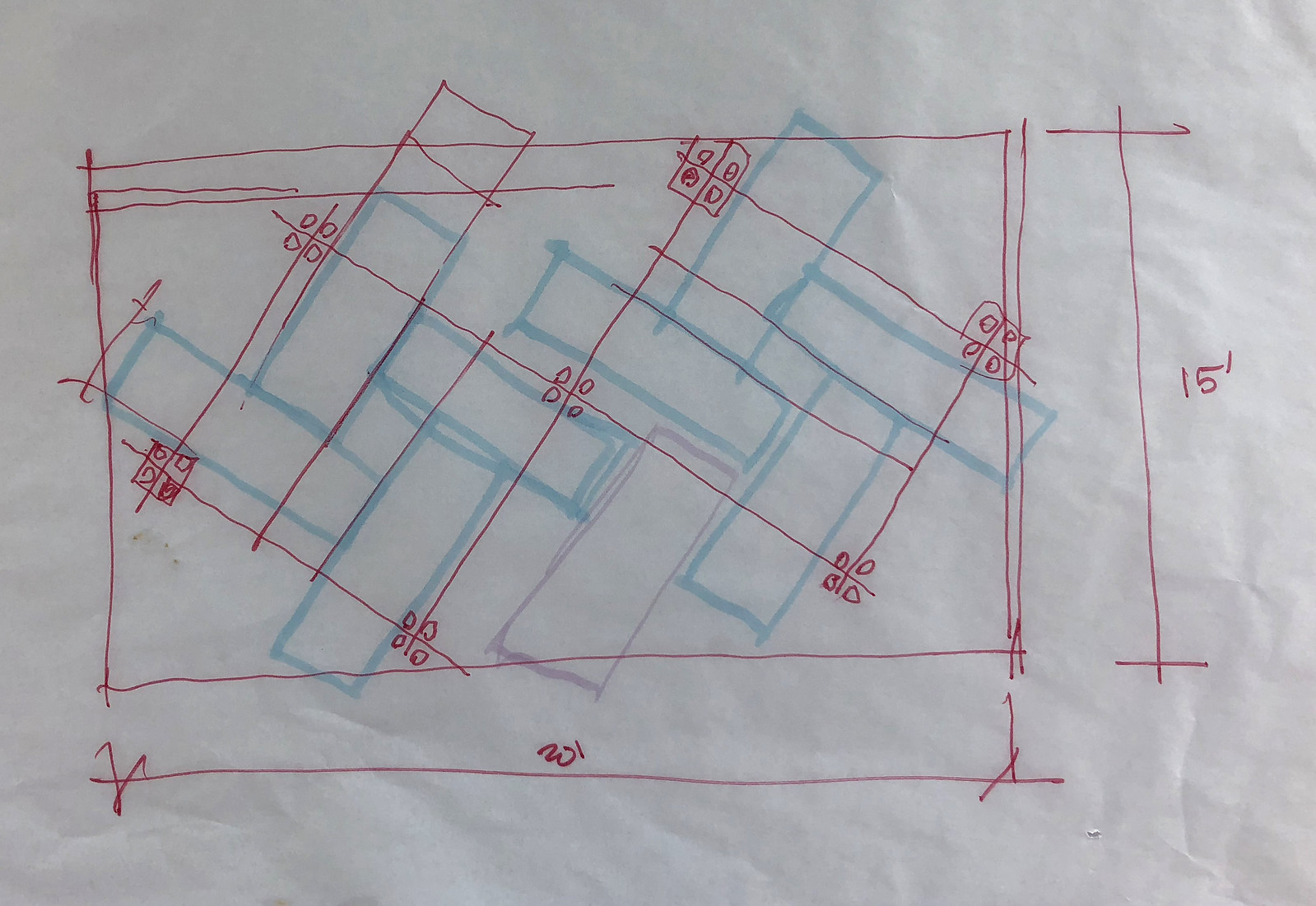This image appears to be a detailed sketch or an abstract art piece. It features a series of four blue squares on the left and four blue squares on the right, all seemingly interconnected. The composition is accented with red ink that traces over and around the blue squares, adding a dynamic contrast. The interplay of the red and blue elements creates an intriguing and visually stimulating pattern. The artwork is simple yet striking, capturing attention with its bold colors and minimalist design.